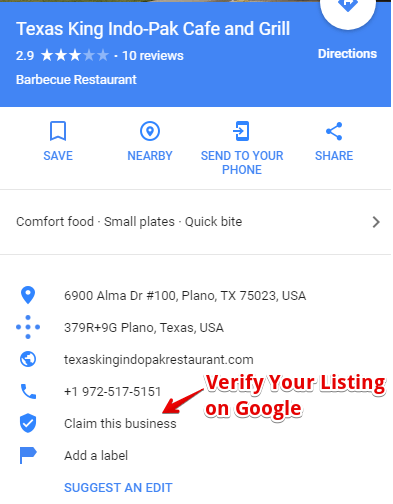**Detailed Description of the Image:**

The image is a screen capture from a mobile device displaying a Google Maps interface. The focal point of the screen is the listing for "Texas King Indo-Pac Cafe and Grill," prominently shown in a blue box at the top of the screen. This restaurant is rated 2.9 stars based on 10 reviews and is categorized as a barbecue restaurant. Below the restaurant's name, there are navigational options including a directional icon with the word "Directions" underneath, suggesting the option to get directions to the location. Other available options include "Save," "Nearby," "Send to your phone," and "Share," indicating various actions a user can take regarding the restaurant listing.

Additionally, the screen displays more specific details about the restaurant, including its address and phone number. Above this information, there is an instructional prompt with an arrow pointing downwards towards the option "Claim this business." To the right of the arrow, there's a note stating "Verify your listing on Google," implying that this screen capture is part of a tutorial or guide for business owners on how to claim and verify their business listings on Google Maps.

The shape and interface elements confirm that this screen capture was taken from a mobile device, adding context that this image is used in a tutorial format to help business owners navigate and manage their online presence through Google Maps.